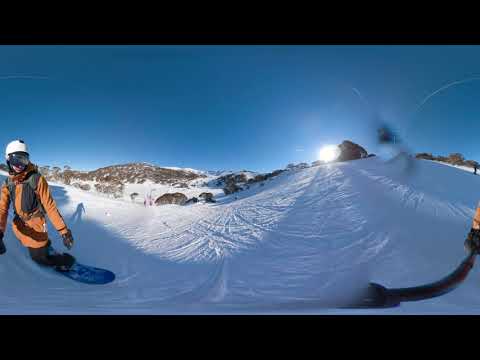In the dynamic photograph, a snowboarder clad in a bright orange ski jacket, black pants, white helmet, and black-frame goggles carves down a snowy mountainside. Mounted on a blue snowboard, he leans into a turn, capturing the exhilarating motion on a selfie stick with a wide-angle lens. The fish-eye perspective emphasizes the snowboarder in the center, making the surroundings appear to stretch outwards. 

Behind him, the sun shines brilliantly, casting a white halo and highlighting the pristine blue sky devoid of clouds, except for a distant trail from a jet airplane. The sun's rays illuminate the scene, creating a vibrant contrast between the snowy slopes and the azure sky. 

In the background, a partially snow-covered mountain and some brown, snow-dusted plants can be seen. The snow is well-trodden with numerous tracks from previous adventurers. To the left, the hill appears covered with forest flora. The atmosphere is crisp and clear, embodying a perfect day for snowboarding. The unique angle of the shot, presumably taken by a GoPro or similar camera attached to a selfie stick, brings a sense of immediacy and presence to the viewer, as if they are right there on the slope.